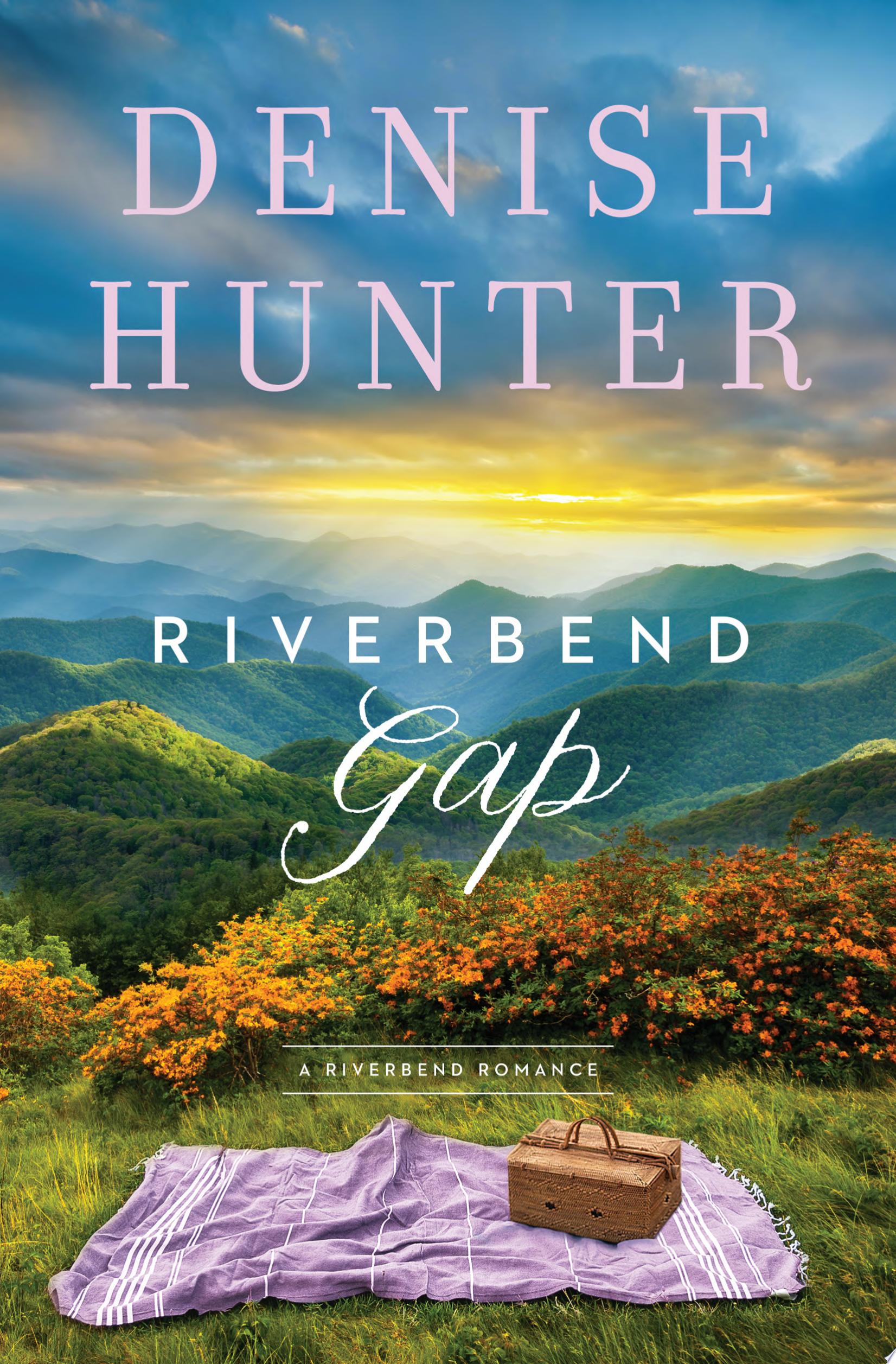The book cover titled "Denise Hunter" prominently features the author's name in large whitish-pink letters at the top, with a subtle hint of pink in the primarily white text. Below this, the title "River Bend Gap" is written in white text, but the word "Gap" is in cursive. Framed by two white brackets, it specifies "A Riverbend Romance." The bottom section of the cover showcases a serene scene: a lush grassy field with a traditional brown picnic basket and a purple blanket adorned with white stripes. From this foreground, the landscape extends into a meadow filled with small reddish-orange flowers among green shrubs, progressing into rolling, green hills that lead to a wide, expansive valley. Overhead, a cloud-covered sky with overcast shades of blue and yellow from the obscured sun casts "god rays" down into the valley, adding a realistic, country feel to the image. The overall style of the cover is lifelike, evoking a peaceful rural environment bathed in natural light.